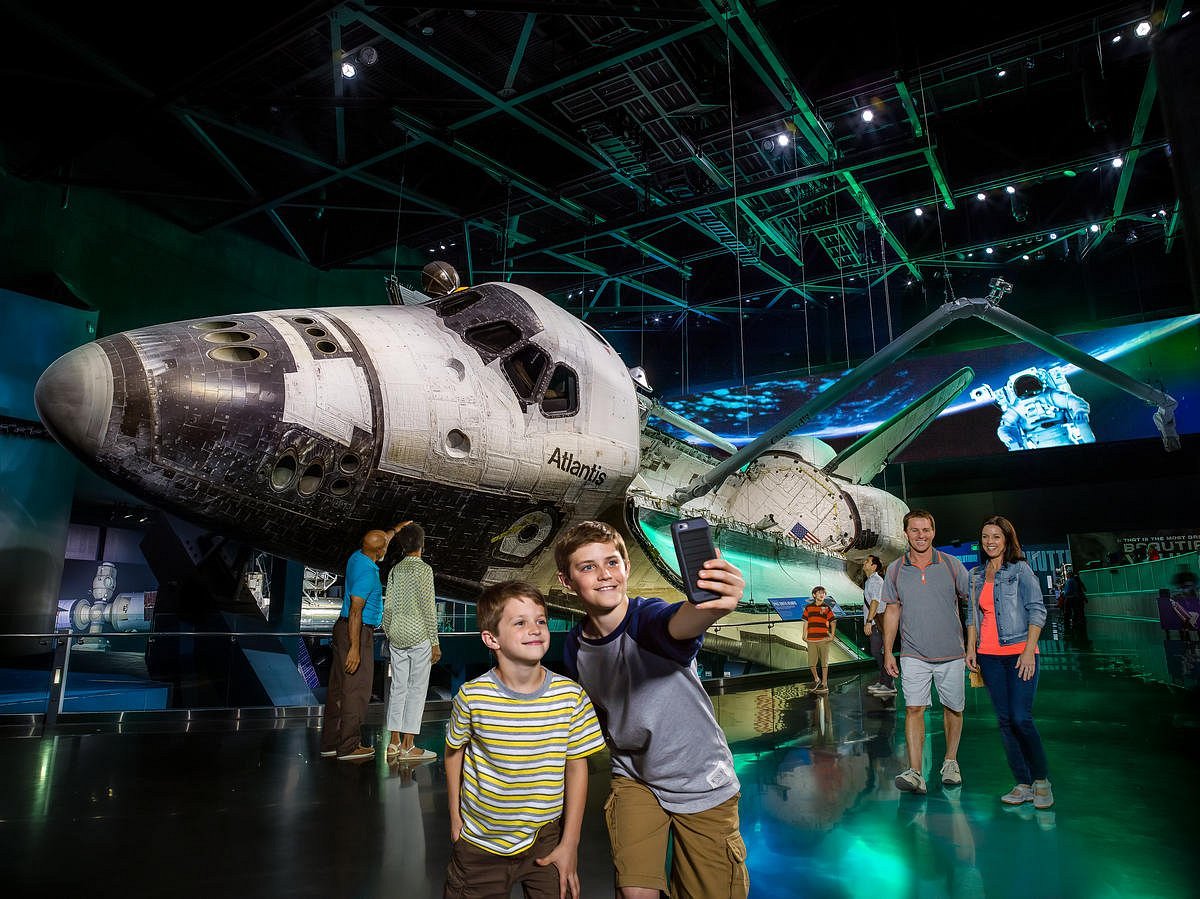The image depicts a bustling indoor space museum or center, set within a large industrial building. Seemingly the focal point of the exhibit, a partially open shuttle labeled "Atlantis" is displayed prominently, allowing visitors to see its black-nosed, white-paneled structure and cockpit windows. The vehicle, tilted for optimal viewing, has green-tinted lighting casting over it from the fixtures hanging along a ceiling replete with metal pipes and wires. 

Directly in front of this majestic shuttle, two young boys take a selfie, their happy faces illuminated by the glow of their smartphone. Behind them, an array of visitors of various ages adds to the immersive atmosphere. To the left, a man points towards the shuttle, explaining its intricacies to a woman who listens attentively. Slightly behind these boys, a couple walks toward the camera, smiling, possibly the boys' parents.

In the far background, a large banner displays an astronaut floating above Earth, giving the scene an authentic space-like ambiance. Below this banner, a man and a boy in a black and red striped shirt stand engrossed in reading an information board about the shuttle. The black reflective flooring adds a layer of depth to the scene, further accentuated by several other displays visible but not as prominent. The overall mood is one of awe and curiosity, with the visuals of astronauts and space images on monitors enhancing the educational experience.